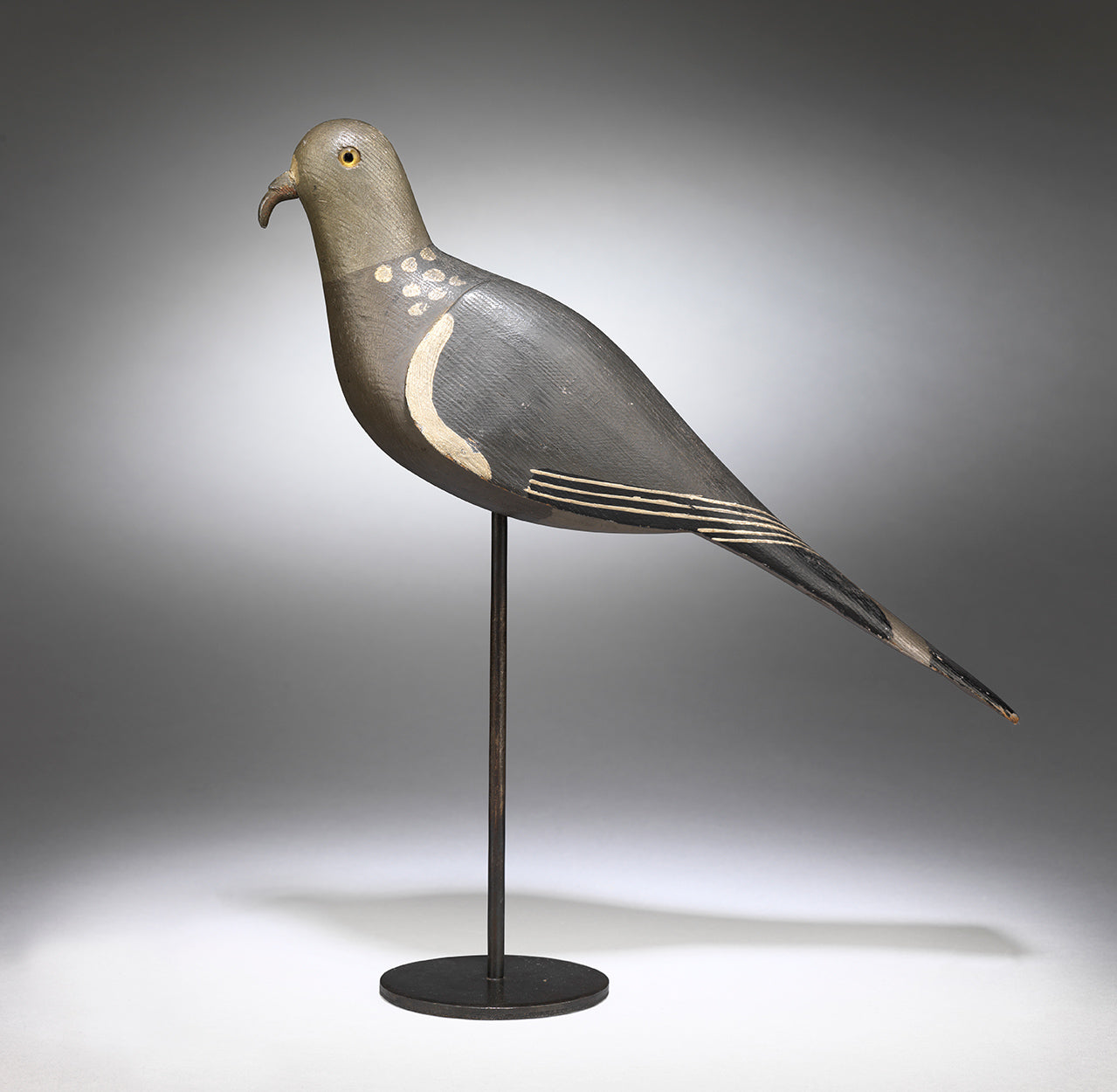The image depicts a wooden sculpture of a pigeon with intricate carved details. The bird, mounted on a long black metal rod that extends to a small circular base, has a distinctive long, slightly curved beak and vibrant orange eyes. Its head and chest exhibit a bronze-brown hue, while the feathers and wings are rendered in darker shades of grey and black. The statue features pale cream-colored stripes along the edges of its wings and tail, as well as white spots on its neck. The background of the image is primarily in various shades of grey, and the bird's shadow is visible against the surface on which it stands.